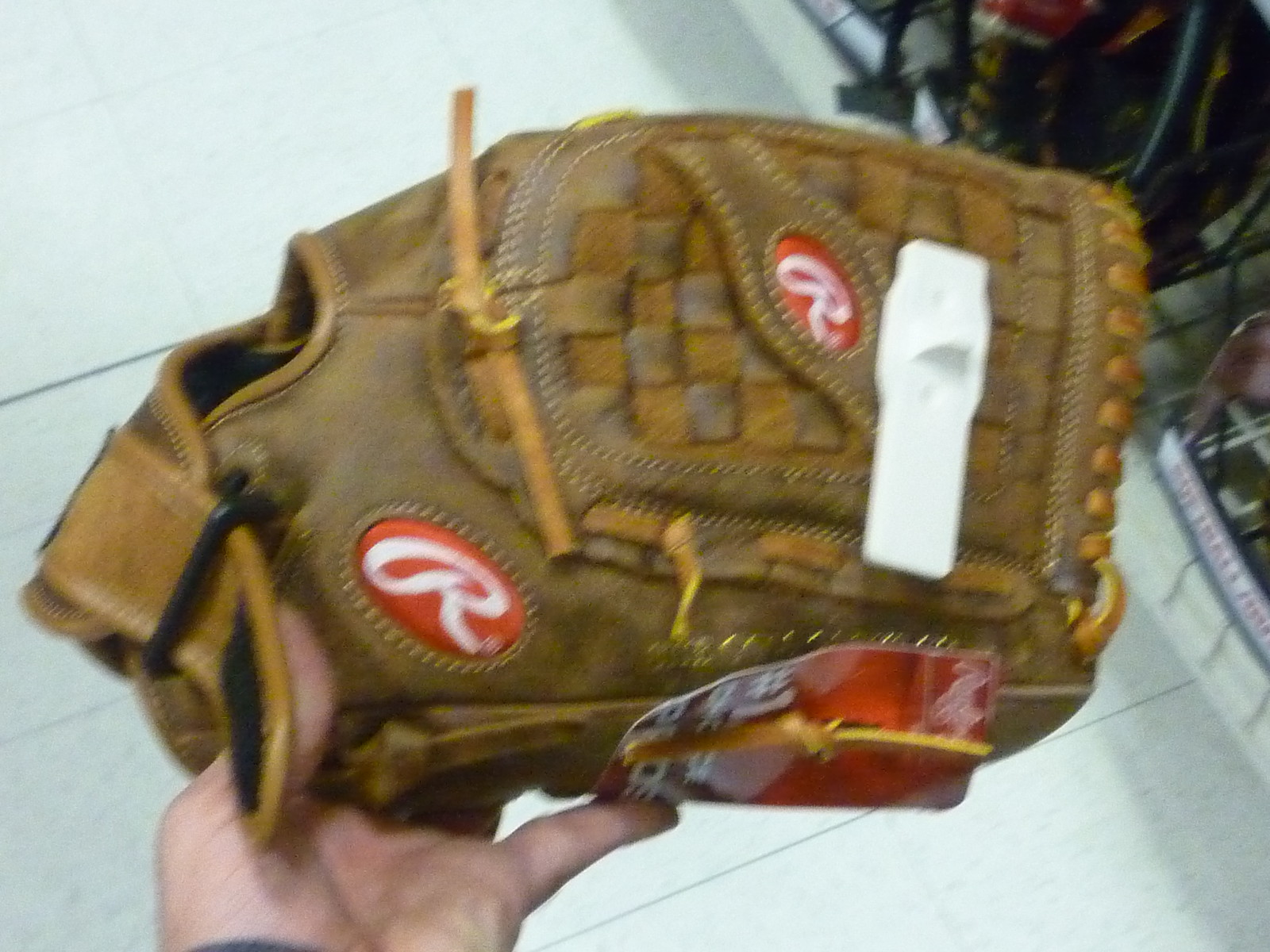A grainy and somewhat blurry photograph depicts a brown catcher's mitt, primarily positioned with the wrist portion towards the left and the glove opening towards the right. The glove showcases a variety of textures, including a prominent crisscross basket weave pattern in its central area. Just above this woven section, there's a distinctive red oval patch featuring a white 'R'. The same red oval patch with the letter 'R' can be found near the wrist, where the glove strap is visible with an open black Velcro portion. Additionally, the glove bears a small red tag and an anti-shoplifting white tag. The mitt is held by a left hand, visible from the wrist down, with the palm underneath the glove. In the background, a white surface is discernible with a scattering of green plants in the upper right corner.